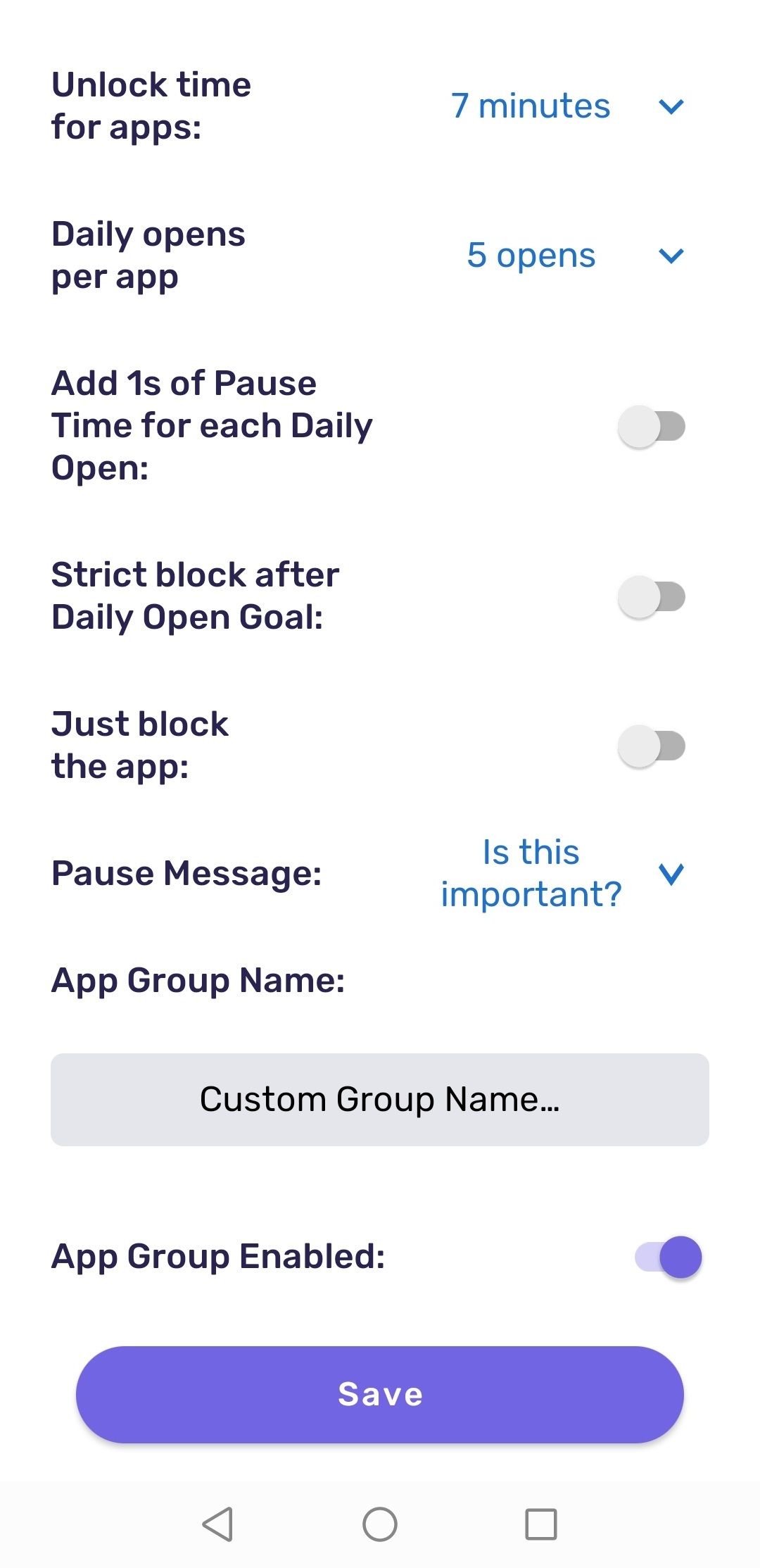This image is a vertically-oriented screenshot set against a white background. In the upper left corner, there is bold, dark blue text that reads, "Unlock time for apps." Adjacent to this on the right, in lighter blue text, it states, "Seven minutes," accompanied by a pull-down arrow. 

Below, you find the heading "Daily opens per app" in bold, dark text. To its right, it mentions "Five opens" along with another pull-down arrow. 

Further down, there is the instruction, "Add one second of pause time for each daily open," with a toggle switch to the right, which is not turned on. Following this instruction, "Strict block after daily open goal" is written, accompanied by another inactive toggle switch to the right.

Continuing downward, "Just block the app" is displayed in bold text with a corresponding toggle switch that is also not activated. 

Next is the "Pause message" in bold text, next to which it asks, “Is this important?” This text is followed by a pull-down arrow.

Towards the bottom, there is the label "App group name" followed by a text box containing the placeholder "Custom group name."

At the very bottom of the image is a blue "Save" button.